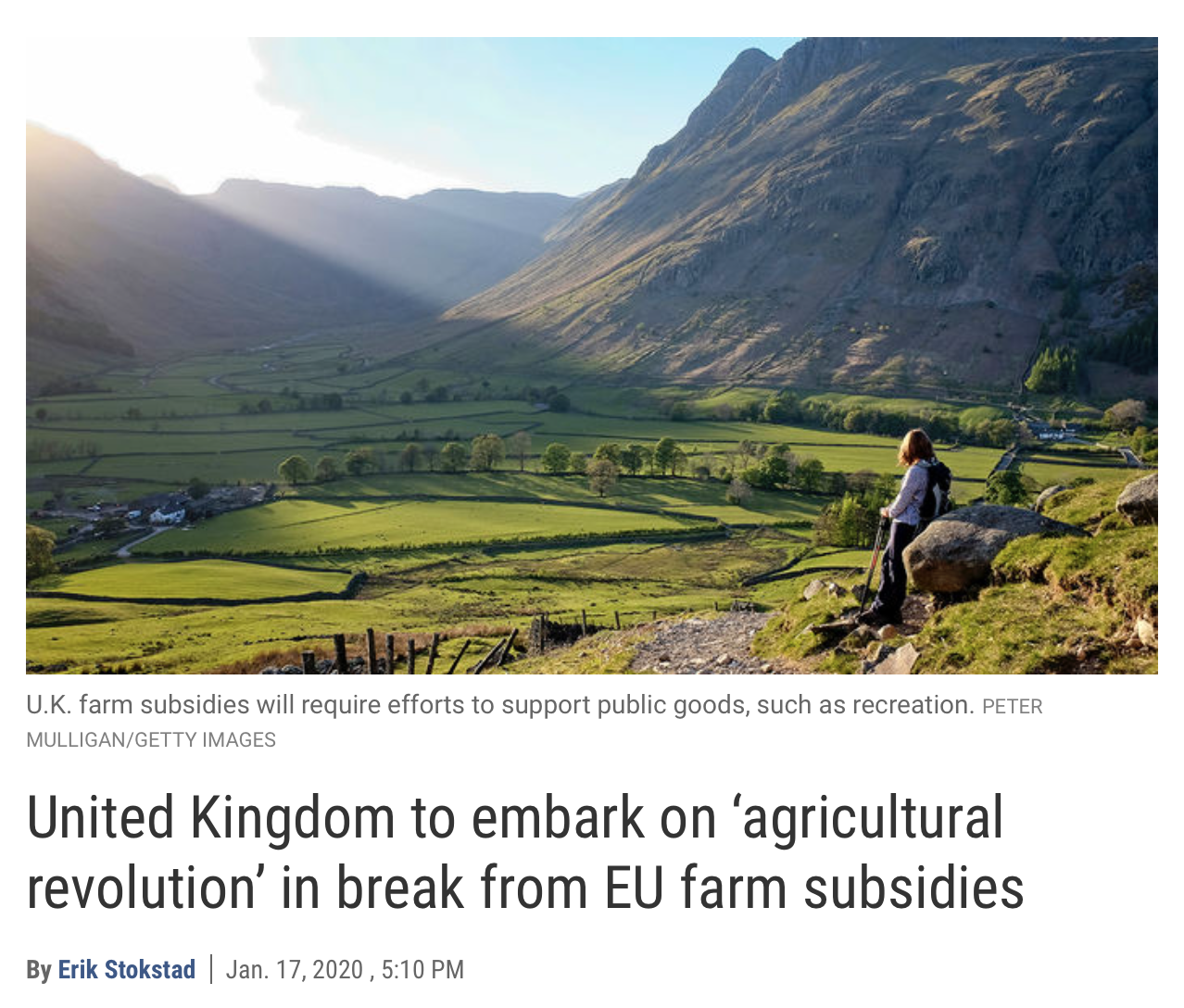A group of hikers is perched atop rugged rocks, overlooking a breathtaking mountain landscape. The scene is a layered vista of mountains that ascend in natural terraces, each level offering a new vantage point. The trail begins at the foot of these formations and winds upwards, flattening out before scaling higher peaks. Bathed in the golden rays of the sun, the lush green valley below is a patchwork of fields, divided by lines of trees and bushes which serve as natural boundary markers. Some old wooden fences, now dilapidated, hint at a long history of land use. One woman stands in the foreground, her head turned to take in the stunning scenery. Equipped with a backpack and a walking stick, she embodies the spirit of adventure and appreciation for nature. The image is captioned with a 2020 headline, "UK farm subsidies will require efforts to support public goods such as recreation. United Kingdom to embark on agricultural revolution and break from EU farm subsidies," reflecting a period of significant policy change.